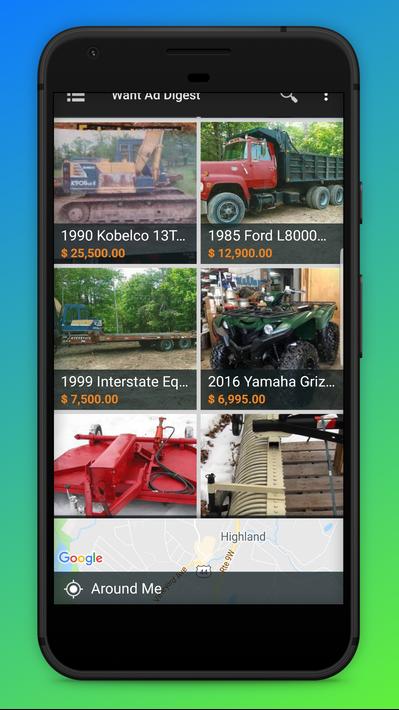This image showcases a black smartphone set against a vibrant background that transitions smoothly from blue at the top to green at the bottom. The smartphone's screen displays six images of various pieces of farm machinery, each accompanied by specific details.

From left to right and top to bottom, the displayed equipment includes:

1. A piece of machinery resembling a backhoe, with no specified details.
2. A 1990 Kobelco 3-ton machine, priced at $25,500.
3. A 1985 Ford L8000, listed for $12,900.
4. A 1999 Interstate ES trailer, offered at $7,500.
5. A 2016 Yamaha Grizzly four-wheeler, green in color, priced at $6,995.
6. Two pieces of farm machinery that appear to be bush hogs, one red, with the price information partly cut off, and the other without visible pricing.

Below the images of the farm machinery, the screen displays a Google Maps view, indicating a location named "Highland." An icon labeled "Around Me" is also visible.

This detailed caption provides a comprehensive description of both the smartphone's screen content and the background details.